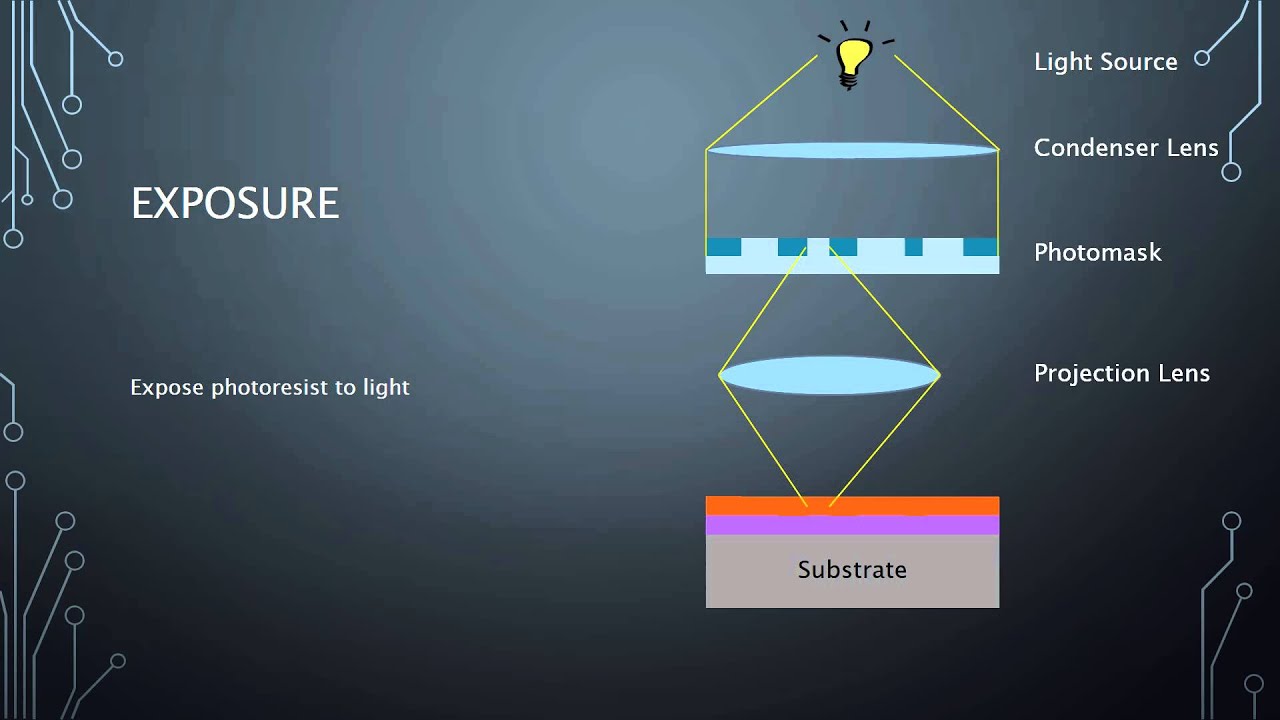The image showcases a detailed diagram on a grey background adorned with electronic circuitry symbols, typical of a circuit board, featuring circles and lines on both sides. The main text, "EXPOSURE," prominently displayed in capital letters, is followed by a directive: "EXPOSE PHOTO RESIST TO LIGHT." At the top, a cartoon light bulb signifies the light source, beneath which lies a series of components essential for the process. These include a lens, an area represented by straight lines and vertical indentations, another lens, and finally, a substrate marked by thin orange and magenta lines, culminating in a substantial greyish-green line labeled "SUBSTRATE." To the right, the diagram details each stage: "Light Source," "Condenser Lens," "Photo Mask," "Projection Lens," emphasizing the path the light takes from source to substrate. The backdrop of the image features a dark greyish-blue hue with faint technological lines and circles, reminiscent of PowerPoint design options.